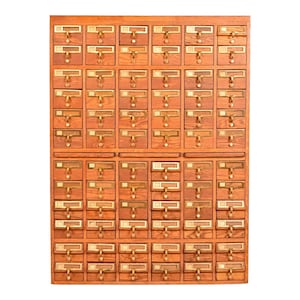This image appears to be a photograph of an old-fashioned card catalog cabinet, typically used in libraries to categorize books using the Dewey Decimal System. The cabinet consists of a grid of rows and columns, specifically 6 columns across and 12 rows, making a total of 72 small drawers. Each drawer is outfitted with brass pulls and square brass label holders, which add to the aesthetic of the cabinet. The wood has an orange-y tint, enhancing its vintage appearance. The image's resolution makes it challenging to determine specific details about the material definitively, yet the overall structure suggests it is a card catalog cabinet, possibly with a secondary function in organizing or securing items. No text or additional context is visible, focusing solely on the intricacy and historical charm of the wooden cabinet with its neatly arranged drawers.